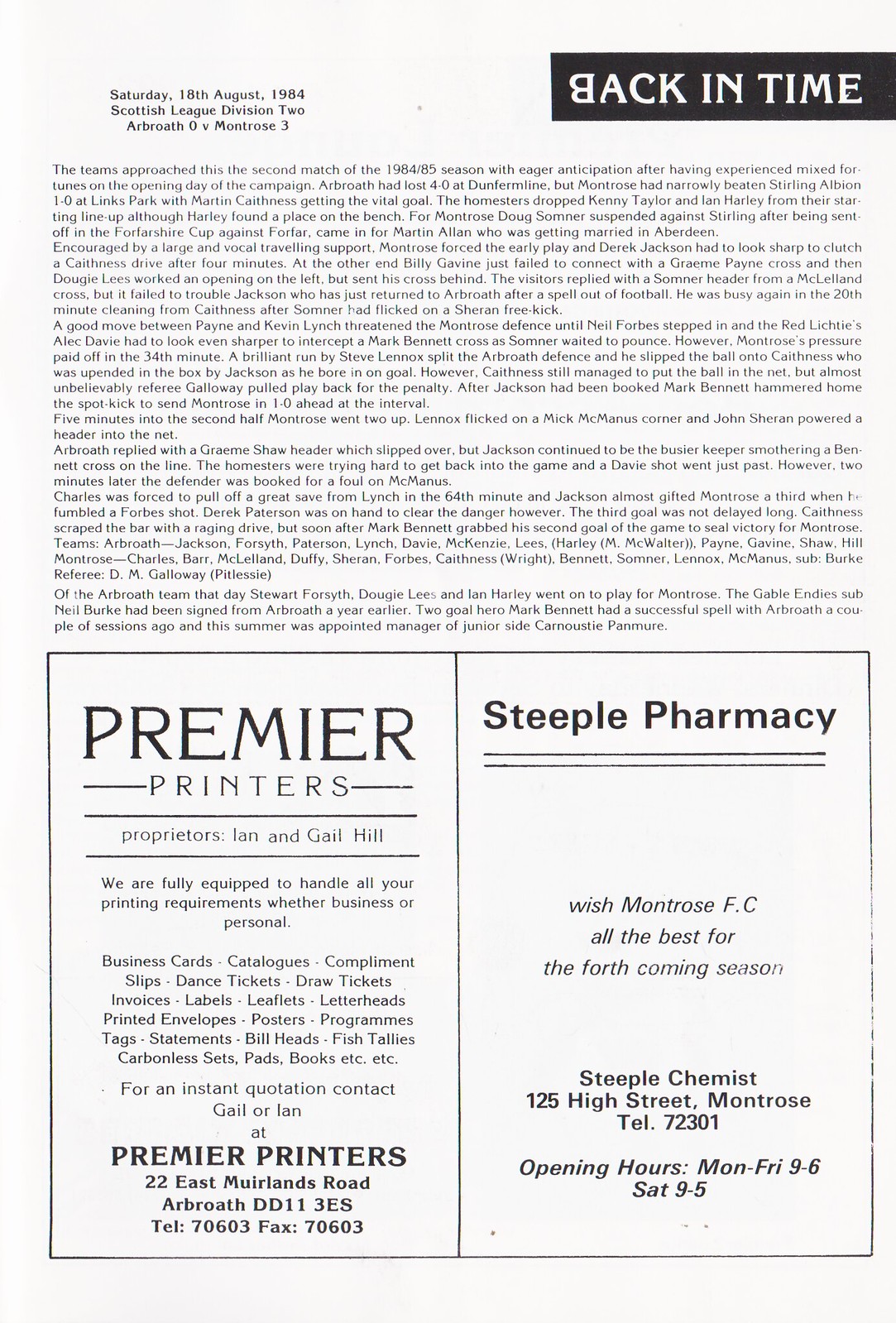The image is a vertically aligned rectangular scan of an off-white piece of paper, predominately in black and white. At the top left, the text reads "Saturday 18th August 1984, Scottish League Division 2, Arbroath 0 versus Montrose 3," providing the date and details of a soccer match between Arbroath and Montrose. In the upper right-hand corner, a black rectangle with white, all-caps text, "BACK IN TIME," catches the eye, with the "B" in "BACK" facing backward. Below this heading, the top half of the page is filled with detailed paragraphs summarizing the events and score of the match. The lower half of the page is occupied by two vertical, side-by-side advertisements. The left advertisement, from Premier Printers, features black all-caps text reading "PREMIER," followed by additional text promoting their printing services for both business and personal needs, listing items like business cards and catalogs. Their contact information is provided at the bottom. The right advertisement is from Steeple Pharmacy, with bold black letters stating "STEEPLE PHARMACY," followed by a message wishing Montrose FC success for the forthcoming season. At the bottom, it lists Steeple Chemist’s address, phone number, and operating hours. The overall image appears to be an old sports pamphlet or report, recapping a soccer match and showcasing related advertisements.